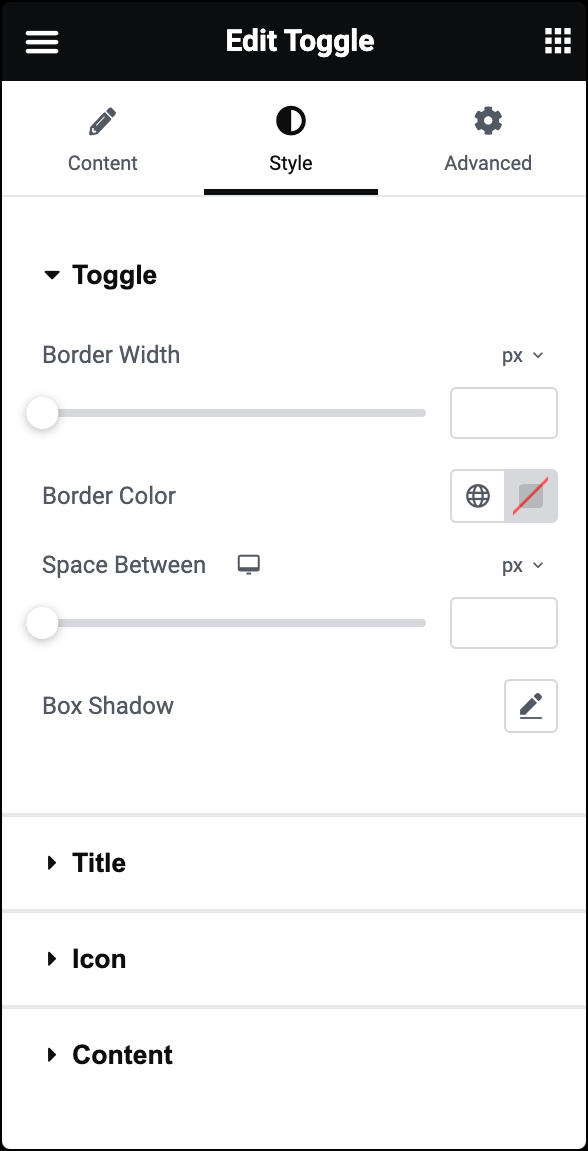The image depicts a screenshot of a settings page. The interface features a prominent black bar across the top with the label "Edit Toggle" centered within it. On the left side of this bar, there is a menu button, and on the right side, a grid button. 

Immediately below the black bar, the rest of the page is white. At the top of this section are three tabs labeled "Content," "Style," and "Advanced." The "Style" tab is currently active, as indicated by its black underline, while the other tabs are in grey.

The left portion of the white section includes a dropdown labeled "Toggle." Below this dropdown is a section for "Border Width," which is controlled by a slider and an adjacent empty field for precise input to its right. Directly above the empty field is a dropdown menu labeled "px" for pixel measurement.

Further down, there's an option labeled "Border Color," accompanied by two buttons aligned to its right. One of these buttons is crossed out in red, possibly indicating a reset or removal option.

At the bottom, there is another slider labeled "Space Between," with an empty field next to it for pixel input, marked with "px," and placed to its right.